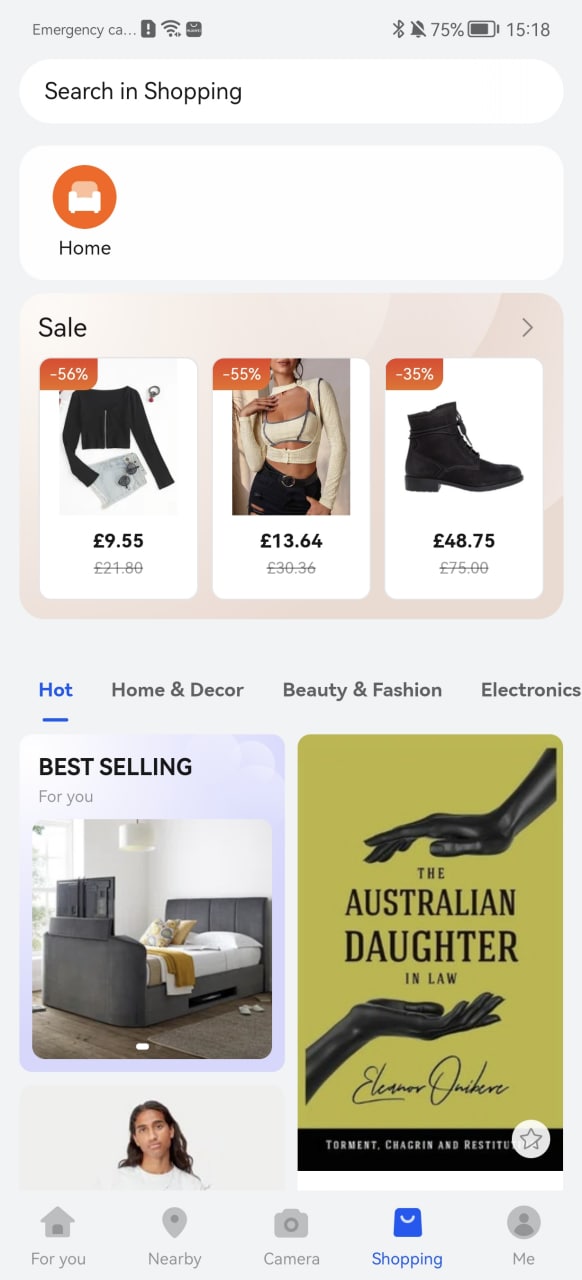An image displays an online shopping interface on a smartphone. At the top left corner, there's a search box with the text "Search in Shopping." Below, a menu features options including "Home," and an orange-highlighted "Search" button with a picture of a couch. Central to the interface is a prominent "Sale" section showcasing three discounted products, each with the percentage reduction in white text on an orange background. 

The first product is a black t-shirt, jeans, and sunglasses combination, discounted by 56%, reducing the price from £21.80 to £9.55. The second product, also clothing, is marked down by 55%, from £30.86 to £13.64. The third item, a pair of black shoes, is 35% off, now priced at £48.75 from £75. 

Below the sale section, categories listed include "Hot," "Home Decor," "Beauty," "Fashion," and "Electronics," with "Hot" highlighted in blue, displaying a "Best Selling for You" banner. Associated is an image of a bedroom setup with a TV stand at the foot of the bed, a text or book on the right-side table, and a book titled "The Australian Daughter-in-law" against a green background with black hands.

At the bottom of the screen, navigation icons include "For You," "Nearby," "Camera," "Shopping," and "Me," with the "Shopping" section currently selected.